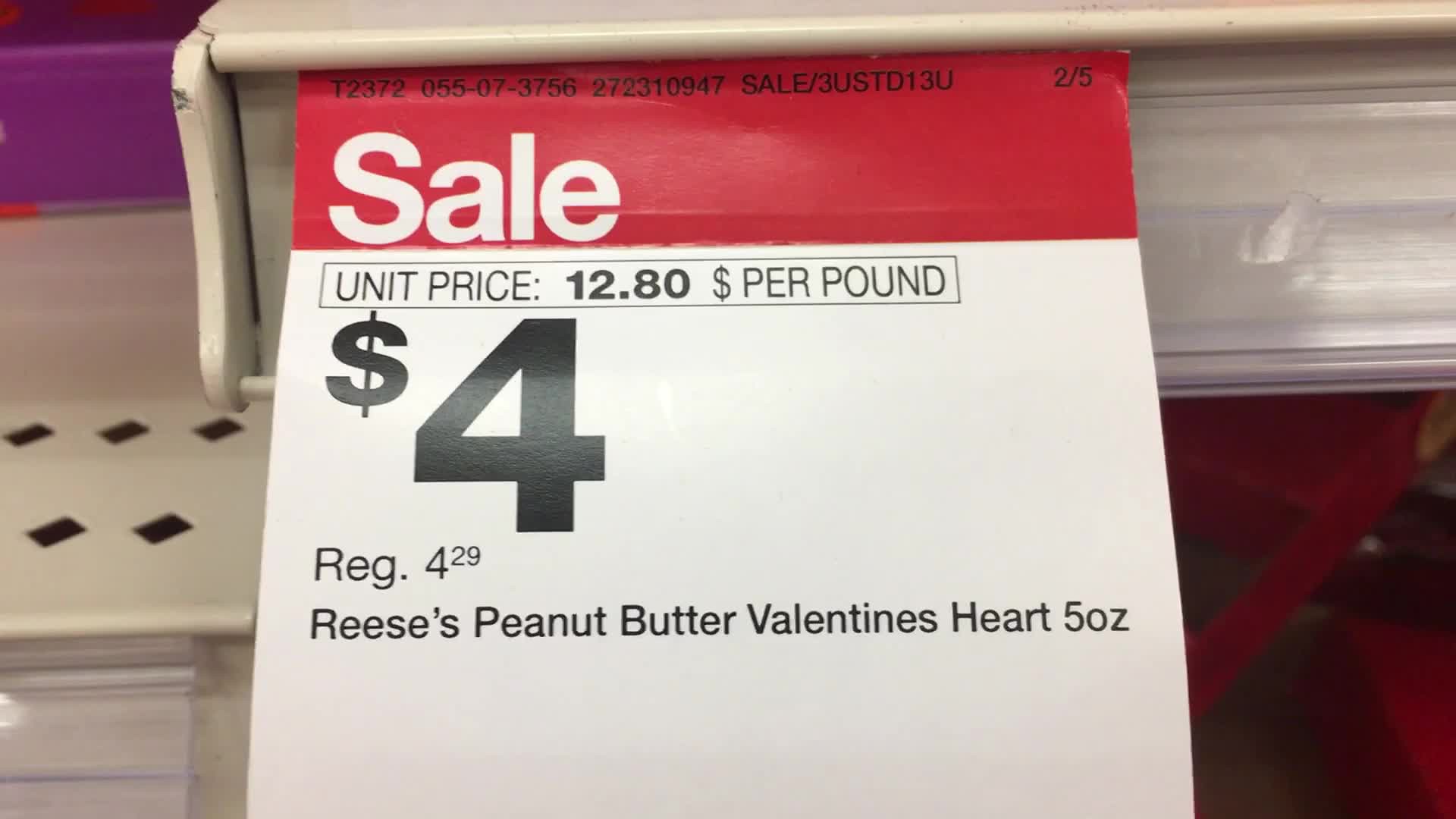This image captures a close-up view of a sales tag attached to the edge of a creamy tan-colored metal shelf, with a red border along the top and a prominent red banner displaying the word "SALE" in white letters. Directly beneath this, the white section of the tag includes detailed product and pricing information. At the top, a set of serial numbers, like T2372055, is printed within the red border. Below, a black-bordered rectangle contains the text "unit price $1280 per pound" in black font. Dominating the center of the tag, a large black dollar sign followed by the number "4" is printed. Just below, in smaller black font, the text "reg 429" indicates the regular price. Further down, the product description reads "Reese's Peanut Butter Valentine's Heart 5oz." The tag, adhered to the shelf's front edge, shows part of another shelf with purple products in the background on the left. Underneath the shelf, partially visible red box-like objects are present. This detailed tag is primarily white and red, with clear, informative black text and is set against the backdrop of the store's shelving system.